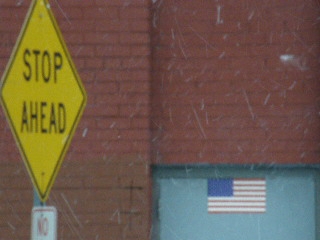This wide-angle photograph, predominantly featuring a red brick wall, is taken from an above-head height perspective along a roadside. Central to the image, the wall is interrupted by a recess, creating an indented section that divides the left protruding part from the right. In the bottom right corner, there is a further recessed light blue door with only its upper portion visible. A small American flag adorns the top center of the door, spanning approximately one-third of its width. On the far left side of the image, a yellow diamond 'Stop Ahead' sign dominates the space, stretching from the top to nearly the bottom of the frame. Below this warning sign is another smaller sign whose inscription is indiscernible. The composition focuses solely on the wall and signage, with no other elements of the surrounding area visible.